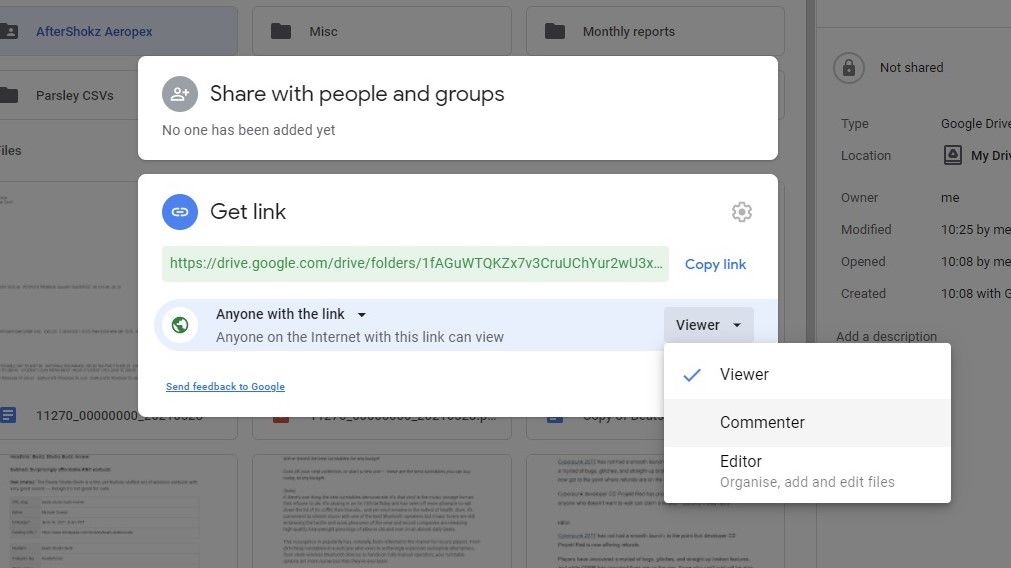The image is a screen capture of a Google Drive interface cluttered with multiple pop-up windows. In the background, the slightly grayed-out Google Drive main page displays a variety of documents and folders. Overlaying this are three distinct pop-up windows:

1. **Top Pop-Up Window:** This small window features a gray circle with an icon of a person and a plus sign, titled "Share with people and groups." It indicates that no one has been added yet for sharing.

2. **Middle Pop-Up Window:** Dominating the screen, this larger window contains a blue circle with a chain link icon, titled "Get link." Below this, a Google Drive URL is highlighted against a green background, followed by the text "Anyone with the link," signifying that anyone on the internet who has this link can view the document. This window suggests a shareable link is active.

3. **Bottom Pop-Up Window:** The third and smallest window is a drop-down menu displaying the sharing permissions. The default selection, "Viewer," has a checkmark beside it. Other options available in the menu include "Commenter" and "Editor," with the latter described as permission to organize, add, and edit files.

Finally, in the bottom left corner of the "Get link" window, a hyperlinked text reads "Send feedback to Google," providing an option to send feedback directly to the Google Drive team.